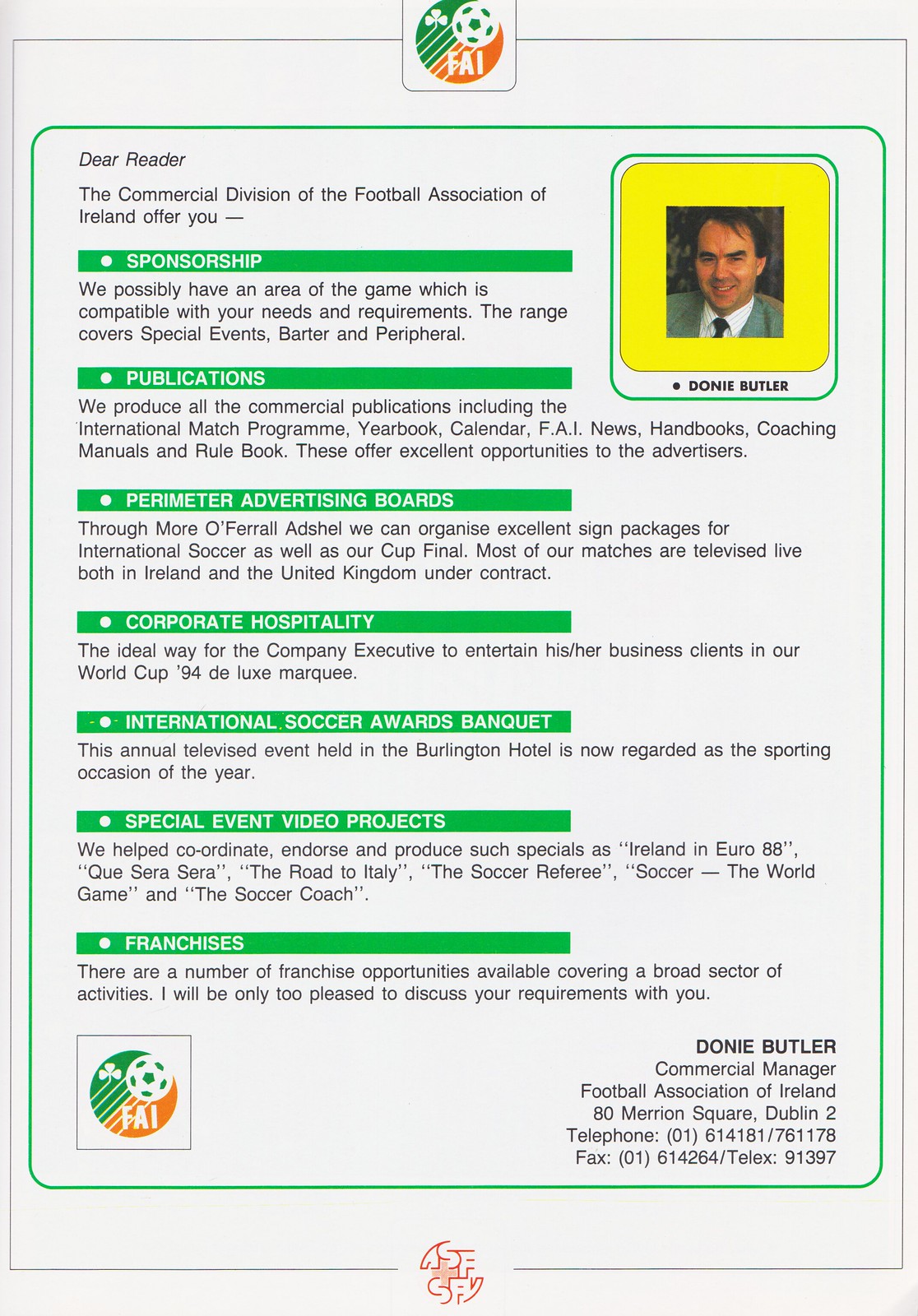This image portrays a promotional brochure from the Football Association of Ireland (FAI) aimed at prospective commercial partners. The backdrop of the page is predominantly white, accentuated by vivid orange and green themes. At the top center and the bottom left corner, the FAI logo featuring a soccer ball is clearly visible, ensuring brand identity.

On the top right-hand side, framed in yellow, is a professional portrait of Donnie Butler with his name captioned underneath in black text. The majority of the text is aligned to the left, structured under various headings highlighted with green backgrounds, white text, and bullet points, detailing sections such as sponsorship, publications, perimeter advertising boards, corporate hospitality, international soccer awards banquet, special events, video projects, and franchises.

Each section expands on how potential partners can benefit. For example, the 'Sponsorship' section discusses matching sponsorship opportunities with the needs and requirements of partners, covering special events, barter, and peripheral engagements. 'Corporate Hospitality' offers prestige through their World Cup 94 deluxe marquee, ideal for business entertainment. Meanwhile, 'Franchises' outlines numerous opportunities across a broad spectrum of activities, encouraging contact for more personalized discussion.

In the bottom right-hand corner, Donnie Butler’s full designation is displayed: "Donnie Butler, Commercial Manager, Football Association of Ireland." His contact details, including address (80 Marion Square, Dublin 2), telephone (01614181761178), fax (01614264), and telex (91397), are provided for further inquiries. This comprehensive and professionally crafted brochure underscores the FAI's commercial offerings and invites prospective partners to discuss mutually beneficial opportunities with Donnie Butler.